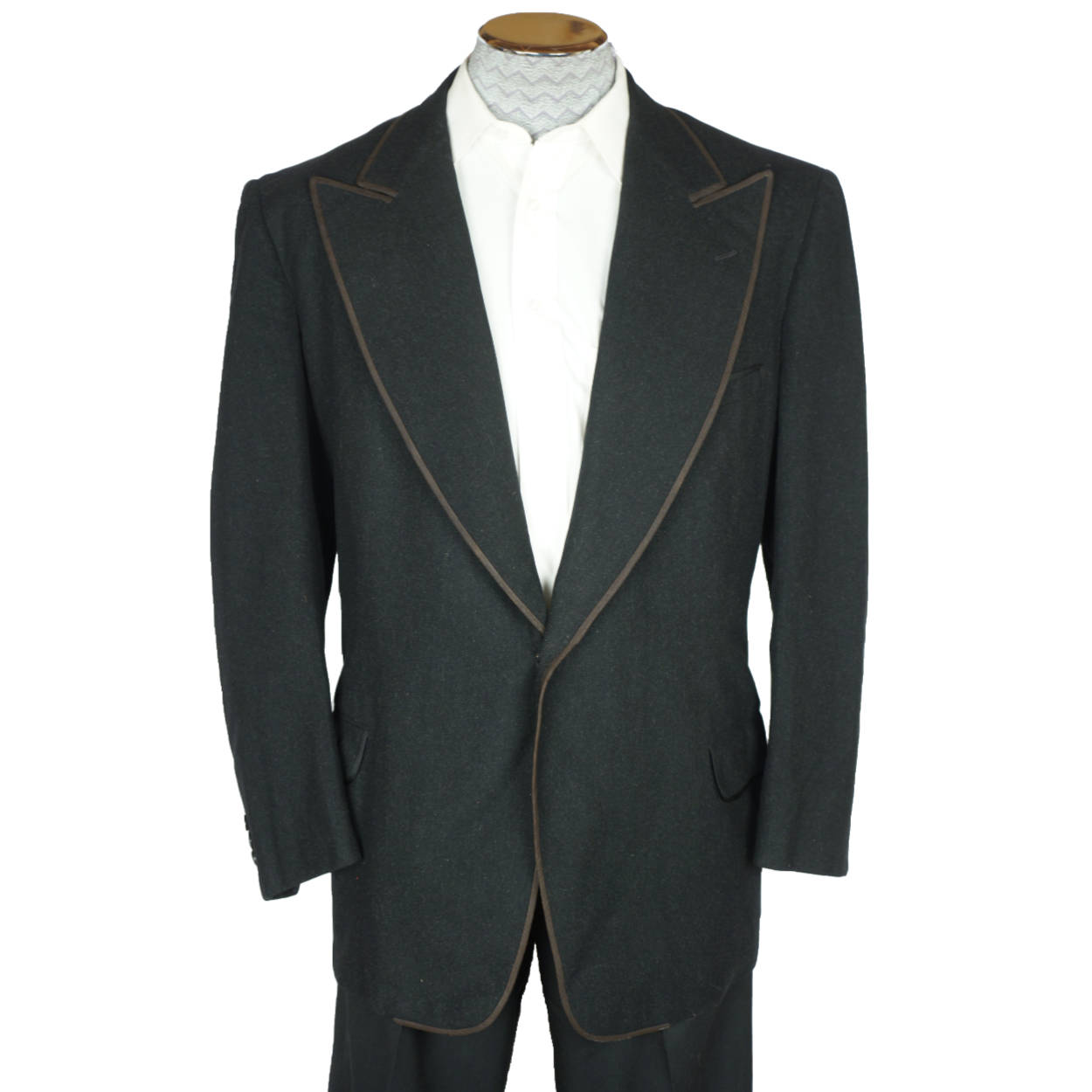The image depicts a sophisticated men's suit displayed on a headless mannequin. The suit is a dark gray, almost black, with subtly intricate brown accent lines along the edges of the jacket. A white button-up shirt, devoid of visible buttons, lies underneath. The mannequin's neck features a textured, white, zigzag-patterned scarf or collar, adding an elegant touch. At the top of the mannequin is a distinct bronze or gold disc. The jacket is complemented with matching gray trousers, visible but cropped at the thigh. The suit jacket boasts a pointed, wide-winged collar and includes a breast pocket on the right side, in addition to two hip pockets. The ensemble is presented against a white background, emphasizing its classic and refined details.